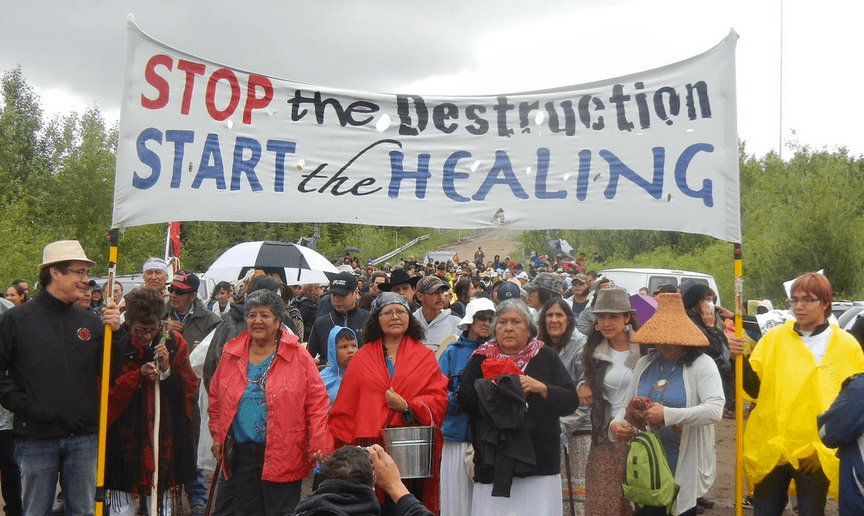In the photograph, hundreds of people have gathered for a protest, holding a large white banner with yellow posts. The banner displays the message, "Stop the Destruction, Start the Healing," with "Stop" written in red text and "Start" and "Healing" in blue text. The words "the Destruction" and "the Healing" are written in black text. The scene is set on a cloudy, potentially rainy day, as many participants are dressed in raincoats, ponchos, and some are holding umbrellas. The banner is held aloft by a person on the right wearing a bright yellow rain poncho and another person on the left in a black sweatshirt or jacket. The crowd features a mix of older women, men, and children, with many older women being prominent at the forefront. Among them, one woman is carrying a bucket and a book bag. A man kneels nearby, taking a photograph of the event. A van is parked on the right side of the dirt path flanked by trees. The group appears to be united in their cause, standing resolutely despite the weather conditions.